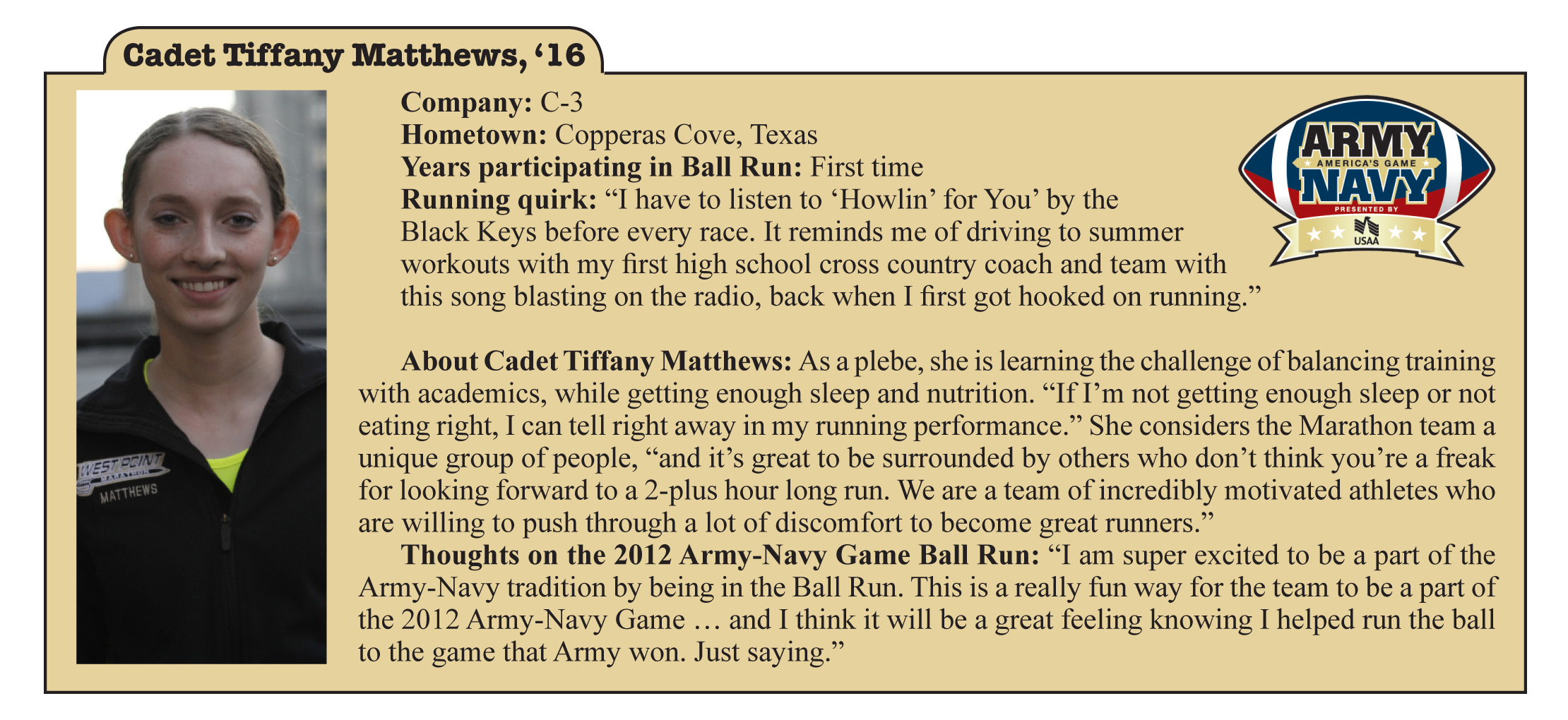The image features Cadet Tiffany Matthews, a member of the West Point class of 2016, who is participating for the first time in the Army-Navy game ball run event. Her profile, prominently displayed, includes a picture of her on the left side, where she is seen with short brown hair and wearing a black West Point fleece, indicating her affiliation with the U.S. Army. Her company is listed as C3, and she hails from Copperas Cove, Texas. The right side of the image contains the text "Army, Navy, America's Game," along with the USAA insurance symbol beneath it. Additionally, the profile includes a personal quote from Tiffany, expressing her enthusiasm about participating in the ball run and mentioning how she listens to "Howling for You" by The Black Keys before every race, a tradition that started during her high school cross-country days.